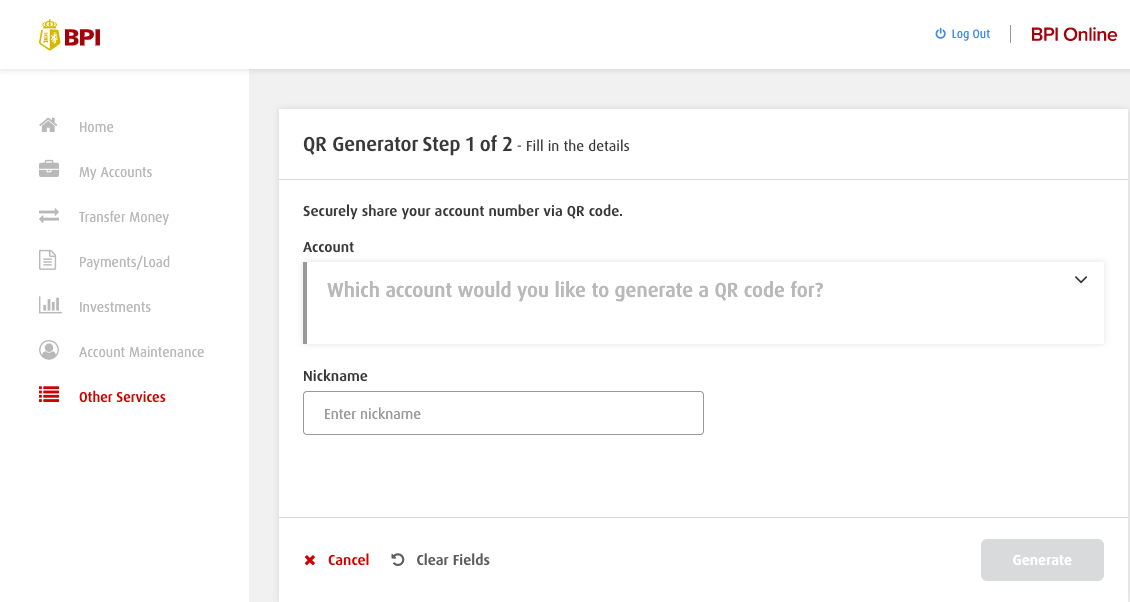The image displays a web page from BPI, identified by its maroon logo at the top that bears a resemblance to the British queen’s crown, indicating that it may originate from Britain. The prominently featured "BPI" is highlighted in a bold, dark font. Adjacent to this, on the right side, are the options "Log Out" and "BPI Online."

On the far left of the page, beneath the logo, there is a vertical menu with several options: Home, My Accounts, Transfer Money, Payments/Load, Investments, Account Maintenance, and Other Services—the latter highlighted in maroon, matching the color of the page header.

Dominating the center is a framed section with a light gray border. It is titled "QR Generator (Step 1 of 2)" with instructions to fill in details to securely share your account number via QR code. The form consists of fields for selecting the account to generate a QR code for and entering a nickname. At the bottom of this section, the buttons "Cancel" and "Clear Field" are available for user input adjustments, while on the right-hand side, a "Generate" button stands ready for action.